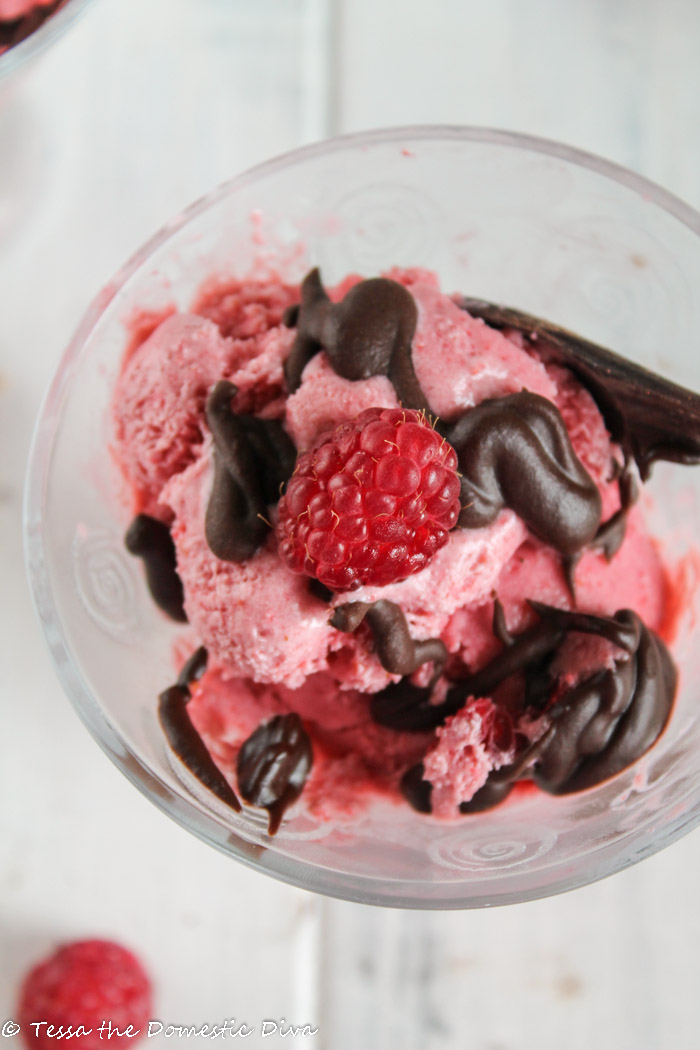This photograph captures an enticing close-up of a pink dessert, possibly a strawberry ice cream or raspberry-flavored sorbet, presented in a small, clear glass bowl with an elegant white swirl design on the exterior. The image, taken from an overhead perspective, showcases the dessert adorned with solidified dark chocolate swirls and crowned by a vibrant, red raspberry. A second raspberry is noticeably placed on the wooden, out-of-focus background, which adds a rustic charm to the otherwise crisp, white setting. Additionally, a small portion of a dark, possibly hand-carved wooden spoon is visible near the top of the bowl. The photo is subtly credited to 'Tessa the Domestic Diva,' visible in the bottom left corner.